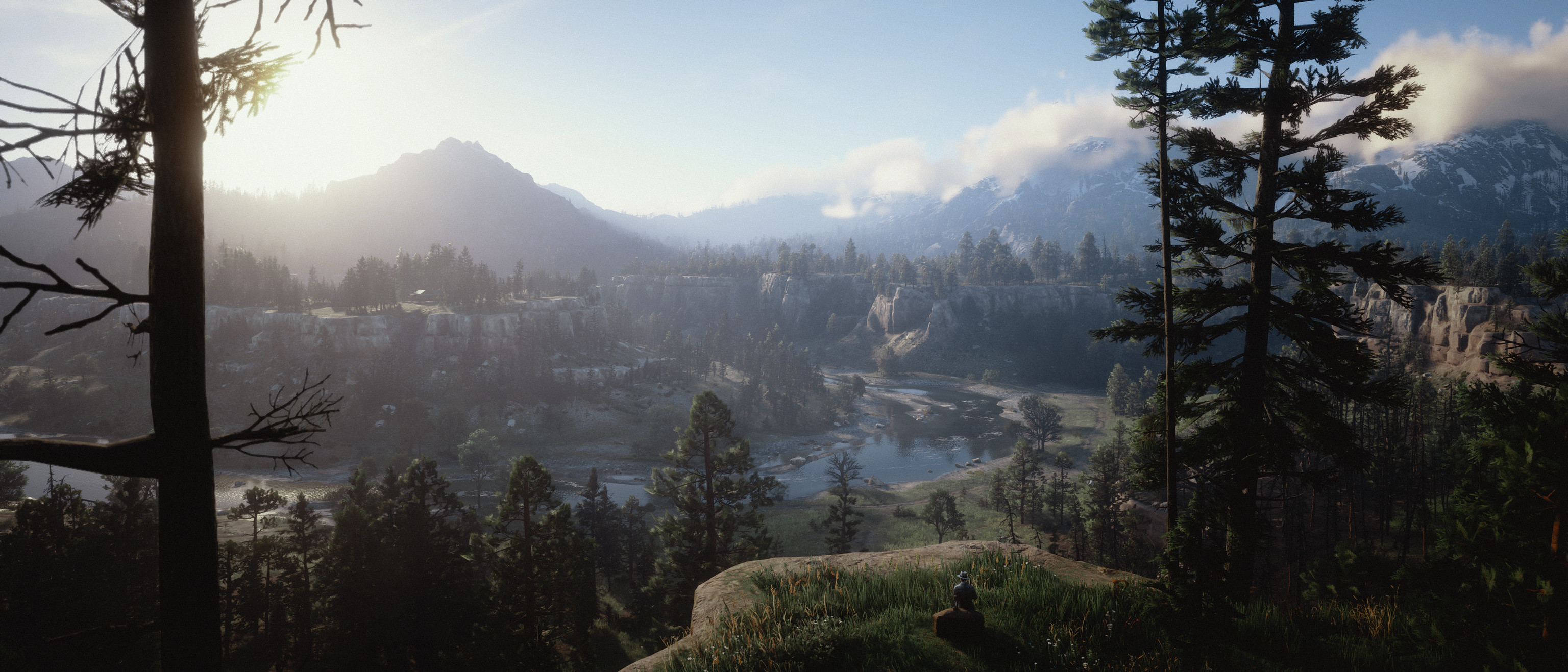A stunningly detailed photo-like digital artwork captures a serene mountainous valley bathed in the gentle light of a rising sun. The sun can be seen peeking over snow-capped mountains in the background, casting long shadows across the landscape. Fluffy white clouds hover around the mountain tops, with some draped across the peaks, contrasting against a clear blue sky. A river or lake meanders through the valley, flanked by patches of lush, green marshland.

In the foreground, there is a rocky cliff with grass, providing a perfect vantage point overlooking the expansive valley. A person-like figure is seated on this cliff, offering a sense of scale and tranquility as they take in the breathtaking view. To the left, a tree with vibrant green leaves stands prominently, while other trees scattered throughout the image display varying degrees of foliage from full to nearly barren. The presence of a stone parapet with what appears to be a balcony-like structure adds a historical or architectural touch to the natural beauty of the scene. Below, a mix of stone hills and large rocky formations are visible, enhancing the rugged beauty of the terrain. Meanwhile, a small bird adds life and movement to this otherwise still and tranquil setting.